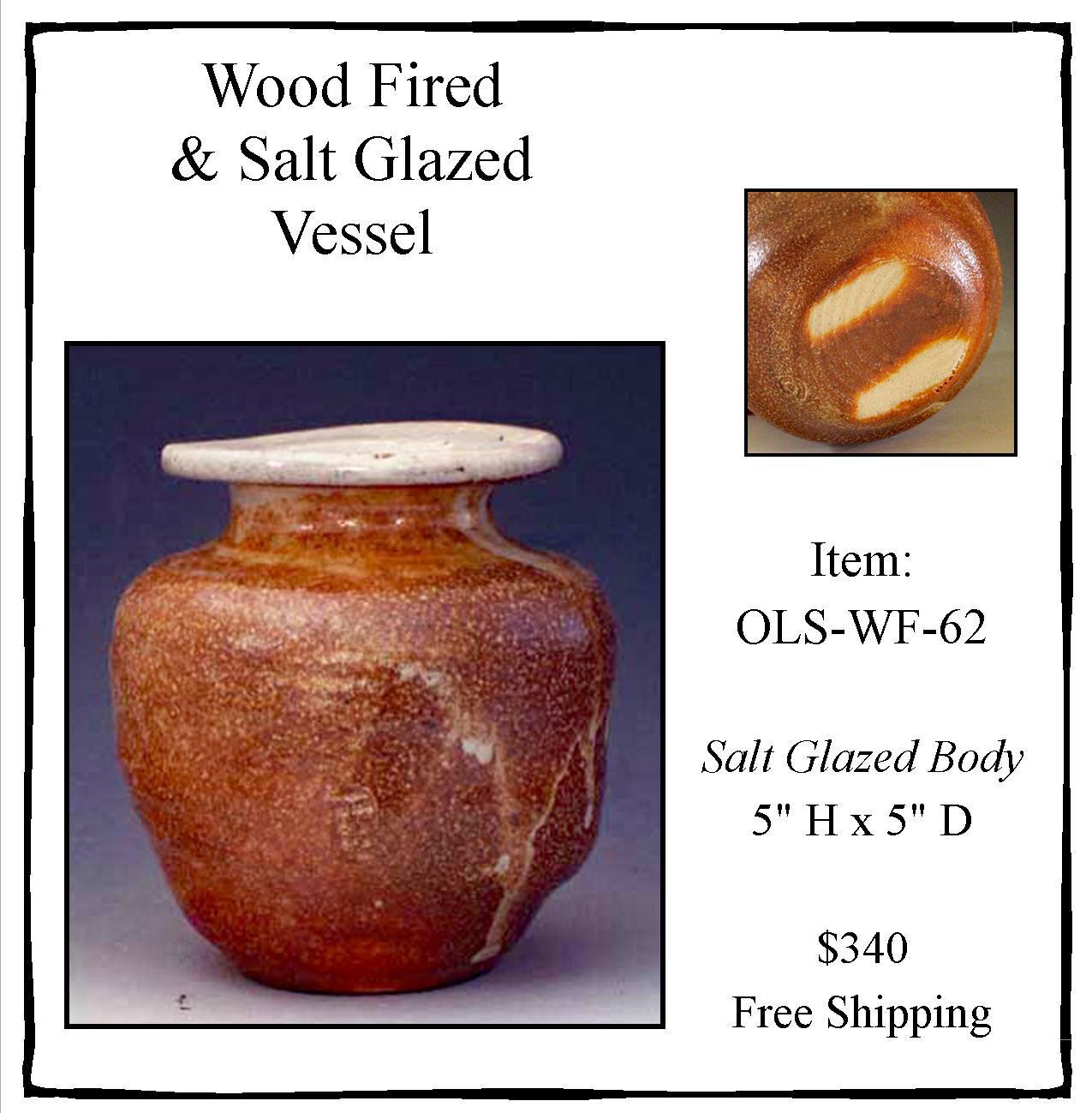The image is a product advertisement for a wood-fired and salt-glazed vessel, identified as item OLS-WF-62. Set against a white background, the advertisement features black text and a black border. The main image, located in the bottom left corner, showcases a side profile of the vase, which has a brown, white, and yellow-speckled body with a flat lighter-colored rim. The smaller inset picture, positioned in the upper right corner, displays the bottom of the vase characterized by a swirling pattern and similar color scheme. The vessel sits against a blue background. Text on the left side of the image reads "wood-fired and salt-glazed vessel." To the right of the inset picture, the text details item specifications: "5H x 5D," "salt-glazed body," and "price: $340 with free shipping."